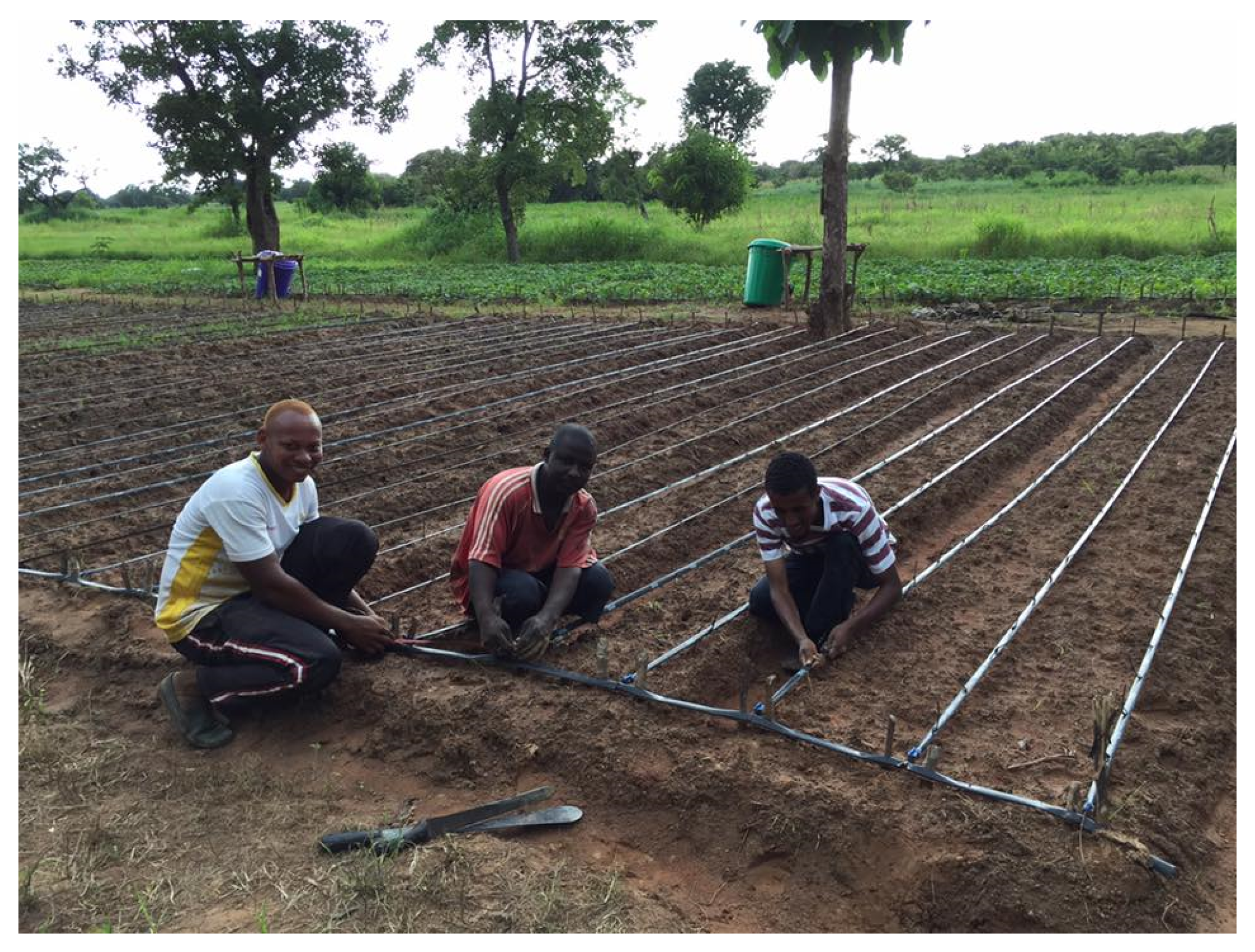This vibrant outdoor photograph depicts three men diligently installing an irrigation system in a field of rich brown soil. The man on the left is dressed in black pants with a white and black stripe down the side, and a white shirt bearing a yellow stripe down the middle. The man in the center wears black pants and a red shirt with white stripes. To the right, the man is focused on his task, donned in black pants and a white shirt accented with brown or purple stripes. All three are crouched on the ground, surrounded by metal tools and pipes, working harmoniously. In the background, a vast expanse of lush green vegetation stretches into the distance, dotted with a few trees and cylindrical bins – one green directly above the men, and another blue one nearby. The bright, clear sky overhead and the distinct lighting emphasize the clarity and vividness of the image, capturing a moment of collective effort and contentment among the men.